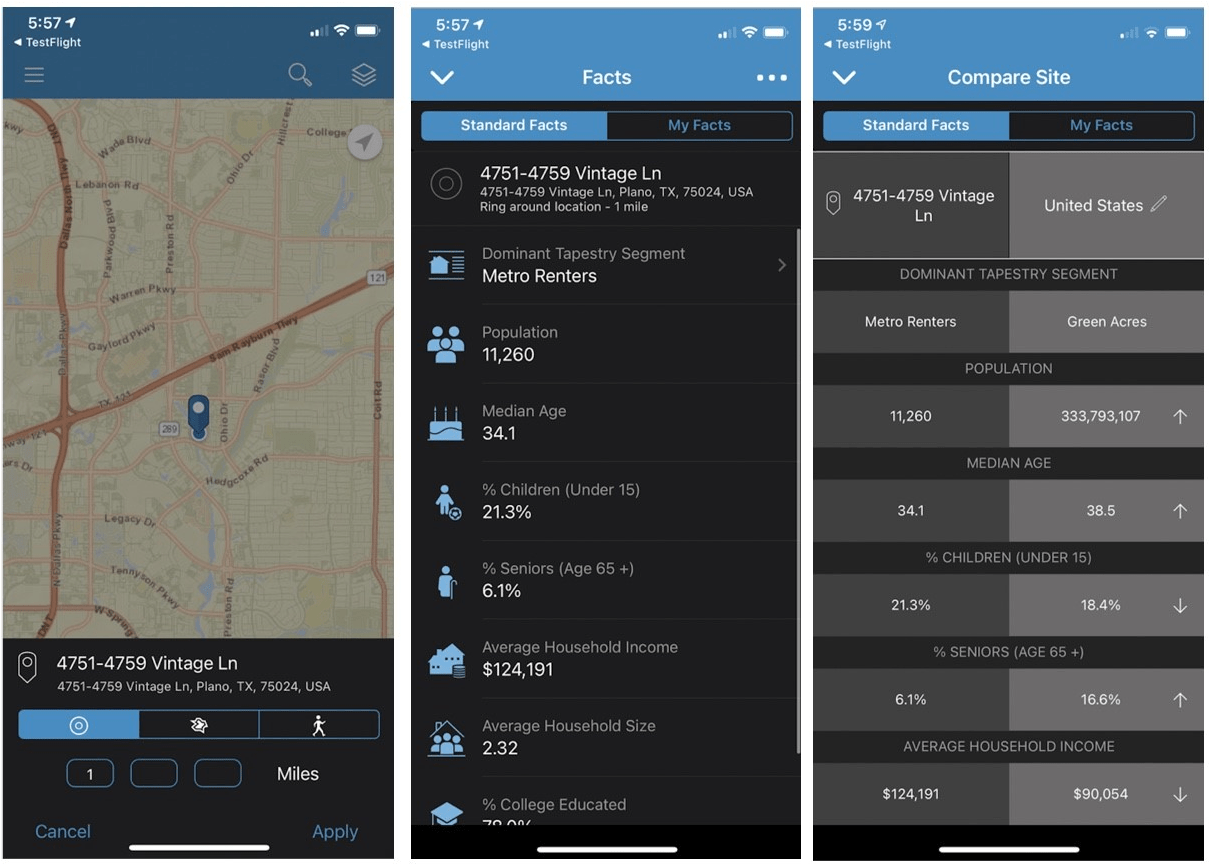**Detailed Caption of Three Tiled Images from a Cell Phone:**

The composite screenshot features three distinct images displayed side by side, showcasing various screens of an app called TestFlight. Below is a detailed description of each image from left to right:

1. **ImageOne:**
   The first image reveals an interactive map interface within the TestFlight app. A single pin is prominently dropped on a location marked "4751-4759 Vintage Lane, Plano, Texas, 75024 USA." This pin likely designates a point of interest or destination. Surrounding the pin are several navigation options, although their exact functions are somewhat unclear. On the left side of the screen, there are two circular icons, one larger and one smaller, possibly represent zoom controls. In the center, there is a slightly ambiguous icon that resembles a bird. To the right is an icon depicting a walking figure, likely for enabling walking directions. Additional control buttons are found at the screen's lower corners: a "Cancel" button on the left and an "Apply" button on the right.

2. **ImageTwo:**
   The second screenshot transitions to a list of detailed statistics about the specified address. The screen presents a title "Facts" with two selectable tabs labeled "Standard Facts" and "My Facts," with "Standard Facts" currently highlighted. Below the address, multiple demographic statistics are displayed. Key details include:
   - Dominant Tapestry Segment: Metro Renters
   - Population: 11,260
   - Median Age: 34.1
   - Percentage of Children (under 15): 21.3%
   - Percentage of Seniors (65+): 6.1%
   - Average Household Income: $124,191
   - Average Household Size: 2.32
   - Percent College Educated: Indistinct, but over 70%

3. **ImageThree:**
   The third image showcases a comparative display of "Standard Facts" side by side with broader statistics labeled "United States." The left section reiterates the aforementioned metrics for the specified address, while the right section provides corresponding national averages. Key comparisons include:
   - Dominant Tapestry Segment: Metro Renters (local) vs. Green Acres (national)
   - Population: 11,260 (local) vs. 333,793,107 (national)
   - Median Age: 34.1 (local) vs. 38.5 (national)
   - Percent Children (under 15): 21.3% (local) vs. 18.4% (national)
   - Percent Seniors (65+): 6.1% (local) vs. 16.6% (national)
   - Average Household Income: $124,191 (local) vs. $90,054 (national)

This comprehensive view across the three images collectively provides a detailed demographic and geographical analysis of the selected address within the TestFlight app.